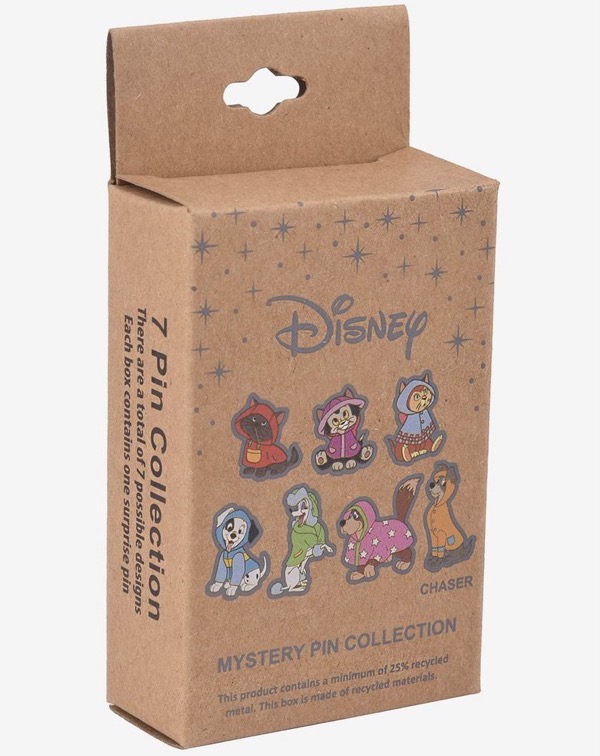The photograph showcases a cardboard box labeled as the Disney Mystery Pin Collection. The front of the box prominently displays the Disney logo, accompanied by the text indicating that it is a Seven Pin Collection with a total of seven possible designs. The box specifies that each box contains one surprise pin and emphasizes its eco-friendly construction, made of recycled materials with a minimum of 25% recycled metal.

The box features images of the collectable pins, illustrating various Disney characters, primarily cats and dogs, dressed in distinctive costumes. The top row displays three cats: a kitten in a red hoodie chewing on the string, a black and white kitten in a pink raincoat adorned with hearts, and a brown kitten in a grey shawl. The bottom row features four dog pins: a Dalmatian in a blue hoodie, an adult cartoon poodle in a green fur coat, a basset hound in a purple rain poncho with stars, and Lady from "Lady and the Tramp" wearing an orange trench coat.

The side of the box reiterates the collection details, with perpendicular text reading "Seven Pin Collection" and further noting that each box includes one surprise pin. Overall, the box combines appealing visuals of beloved Disney characters in whimsical attire with an environmentally conscious message.